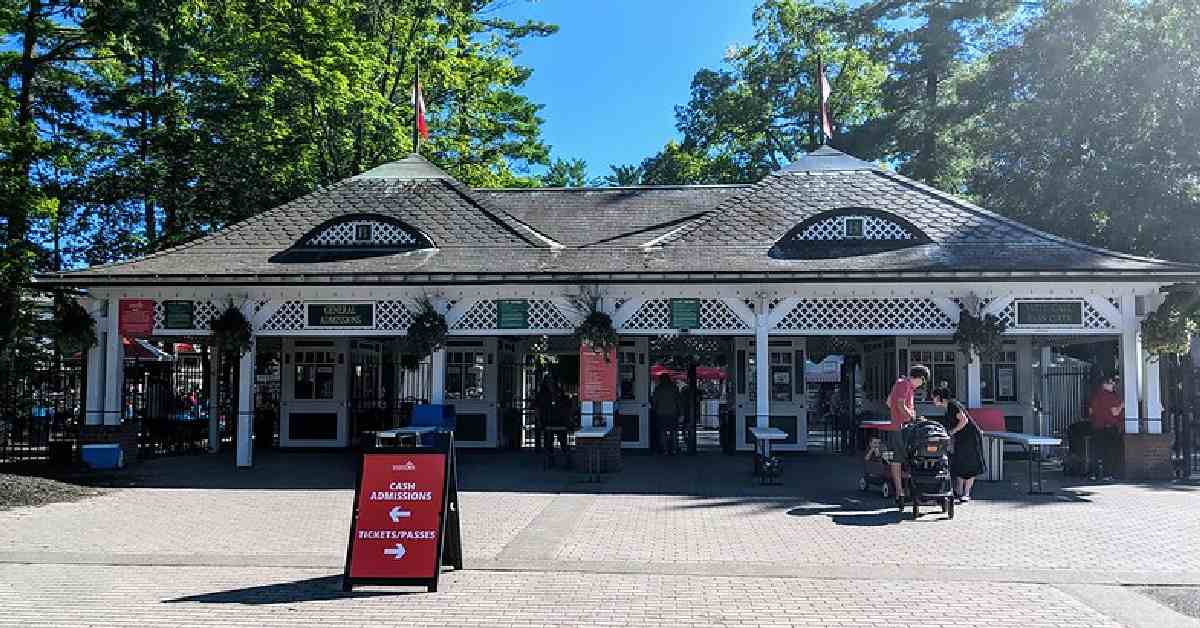This detailed photo captures the entrance to what appears to be an amusement park or zoo. The primary structure is a large, mostly white building with a black, fish-scale tile roof featuring two peaked sections topped with flags. A vibrant blue sky and lush green trees form the backdrop. The entryway, lined with white columns and a lattice top front, has prominently visible white and green ticket booths. A foldable red sign with white text directs visitors: "Cash Admissions" with an arrow to the left and "Tickets and Passes" with an arrow to the right. The foreground features a bright, sunlit, white pavement, with various people, including a couple with a stroller, assembling near the security entrances and ticket booths. There are a few security lines and tables positioned for checking, and on the left, a brick plaza adds a touch of texture to the scene. The atmosphere suggests a welcoming and organized entrance area for visitors.